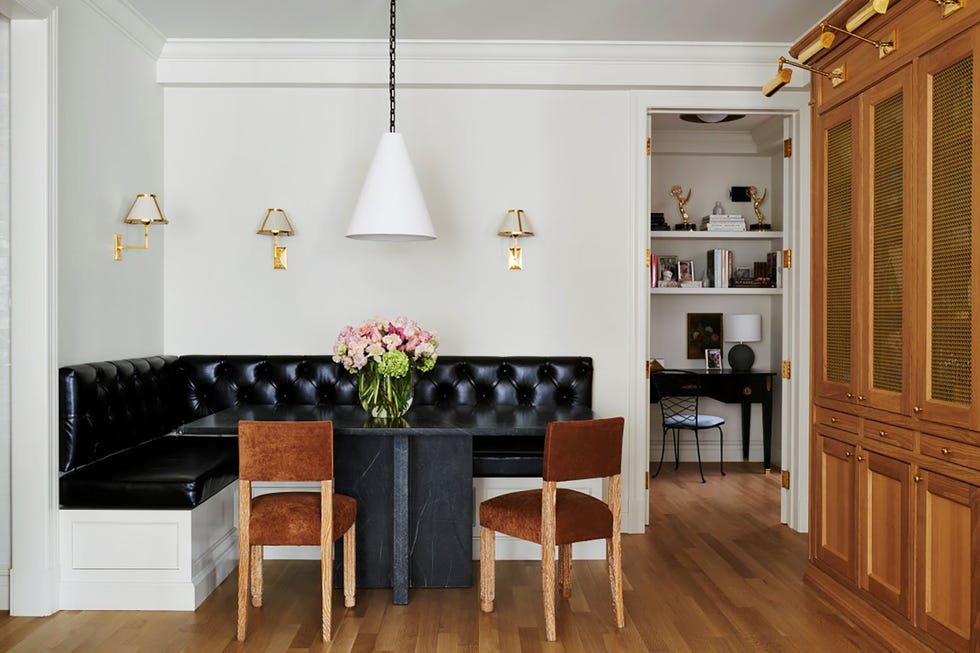This image showcases a cozy interior of a home, focusing on a corner dining area with booth-style seating. The seating features a black leather cushion with a white base, arranged along two intersecting walls. Above the booth hangs a white, cone-shaped light fixture, casting a gentle glow over the scene. At the center of this setup is a black table with a vase of flowers, flanked by two brown chairs on the opposite side of the bench.

To the right, a series of brown cabinets with drawers extends from floor to ceiling, adding warmth and storage to the room. The floor is covered in rich, brown hardwood, contributing to the inviting atmosphere. In the background, there is a black desk accompanied by a black chair. Above the desk, two levels of shelves display various items, including several books, framed photos, and two trophies, suggesting personal achievements. The overall ambiance is both elegant and lived-in, blending practical furniture with personal touches.